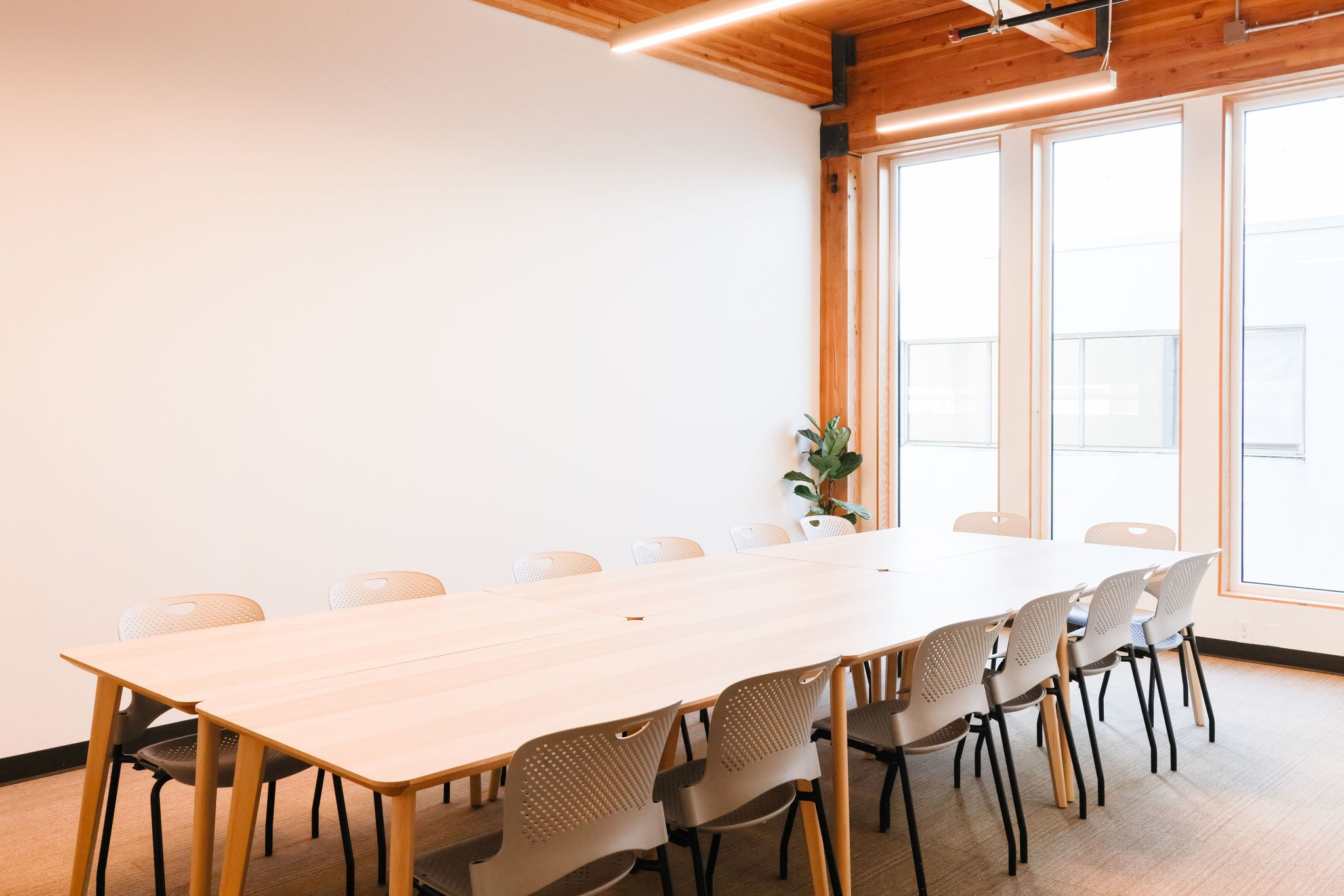The photograph showcases a spacious room likely serving as a conference area, featuring a strikingly large, rectangular table made of light wood, approximately four times longer than its width. The table, which appears as if two long tables have been combined, rests on slightly darker wooden legs and is surrounded by a total of 14 light gray chairs with brown or black legs, arranged with six on each side and two at the head. The room is characterized by an abundance of natural light filtering through three tall, floor-to-ceiling, glass-pane windows that are unobstructed by any blinds or curtains. A plain white wall stands opposite the windows, with the ceiling lined with wooden paneling extending from above the windows. The far corner of the room features a tall, vibrant green plant, about two feet in height, adding a touch of nature to the minimalist setting. The room is accentuated by a blend of colors including brown, black, white, and hints of pinkish and orange hues, with one light visibly turned on, suspended from above, enhancing the clean, airy ambiance.